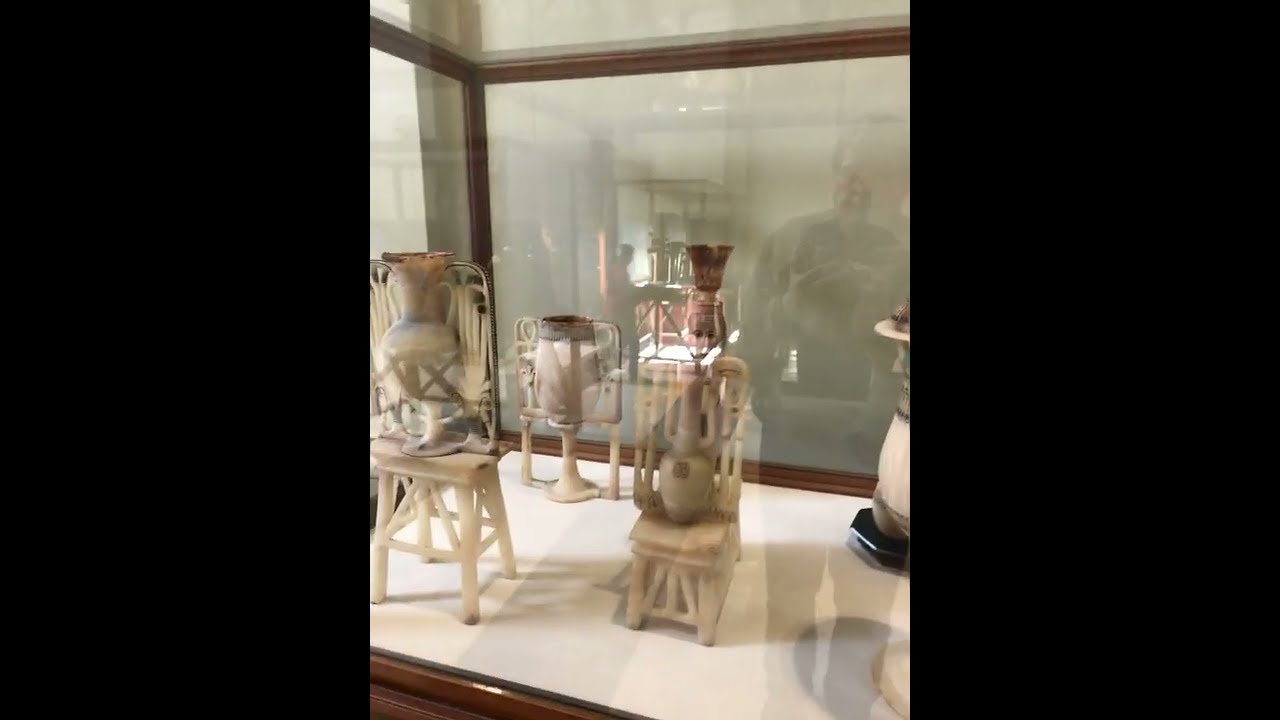This horizontally aligned, rectangular photograph appears to be taken inside a gallery or museum, capturing a display case with a white floor. The case contains four objects, resembling vases or pots, crafted from stone and exhibiting natural colors like whites, tans, and grays. Behind these items, there is a wooden frame surrounding a window, which reflects the image of a person taking the picture. This reflection reveals a man holding either a camera or a phone in front of him, though the details are somewhat blurred. The photograph is flanked by thick, vertical, solid black borders on either side, giving the central image a grayish appearance in contrast. Notably, the image is slightly blurry, suggesting motion when the picture was taken.